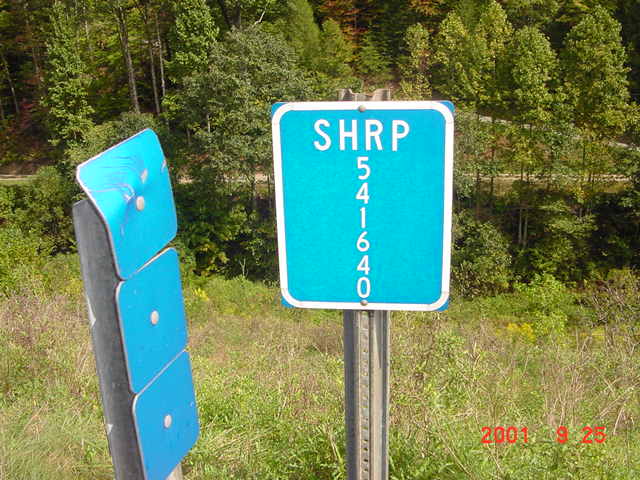This is an outdoor photograph featuring two prominent road signs. The central sign is a blue, square-shaped sign with a white border mounted on a grayish signpost. At the top, it has the white capital letters "SHRP," and below that, the number "541640" is displayed vertically in the same white font. To the left of this main sign, there are three smaller, square-shaped signs of the same blue color, each with white centers, aligned vertically and pointing to the right. They are attached to the same post. The background showcases a landscape of tall, light green and slightly brown grass with some weeds interspersed. Further back, there are trees with green leaves, including a mix of deciduous and pine trees. In addition to the natural scenery, a winding gravel road traverses the entire image, ascending an incline. In the bottom right corner of the photograph, red text indicates the date "2001-925."